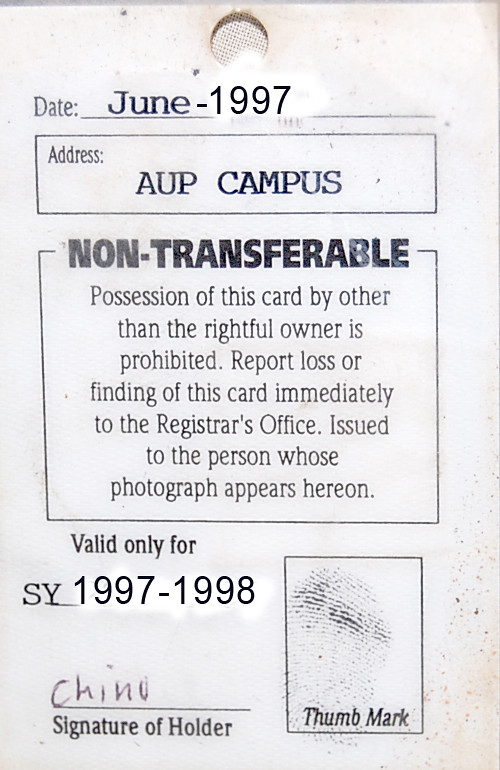The image features a white identification card prominently occupying the background. At the top of the card, the date "June-1997" is typed in bold. Beneath this, an address labeled "AUPCAMPUS" in bold uppercase text appears within a rectangle. Below this is a larger square containing several blocks of text. At the top of the square, the word "NONTRANSFERABLE" is displayed in extra-bold uppercase. Under this are warnings and instructions: "POSSESSION OF THIS CARD BY OTHER THAN THE RIGHTFUL OWNER IS PROHIBITED. REPORT LOSS OR FINDING OF THIS CARD IMMEDIATELY TO THE REGISTRAR'S OFFICE. ISSUED TO THE PERSON WHOSE PHOTOGRAPH APPEARS HEREON." Following this, the card states "VALID ONLY FOR SY-1997-1998" in bold numerals. Below the validation text, there is a line labeled "SIGNATURE OF CARDHOLDER" with the name "CHINO" signed above it. To the right of the signature, a box marked "THUMB MARK" in bold caps contains an image of a fingerprint. The card predominantly features colors of black, white, tan, and gray and appears to be issued by an academic institution, suggesting special permissions or access granted to the cardholder. Some elements, such as the date and validation period, appear to have been edited.